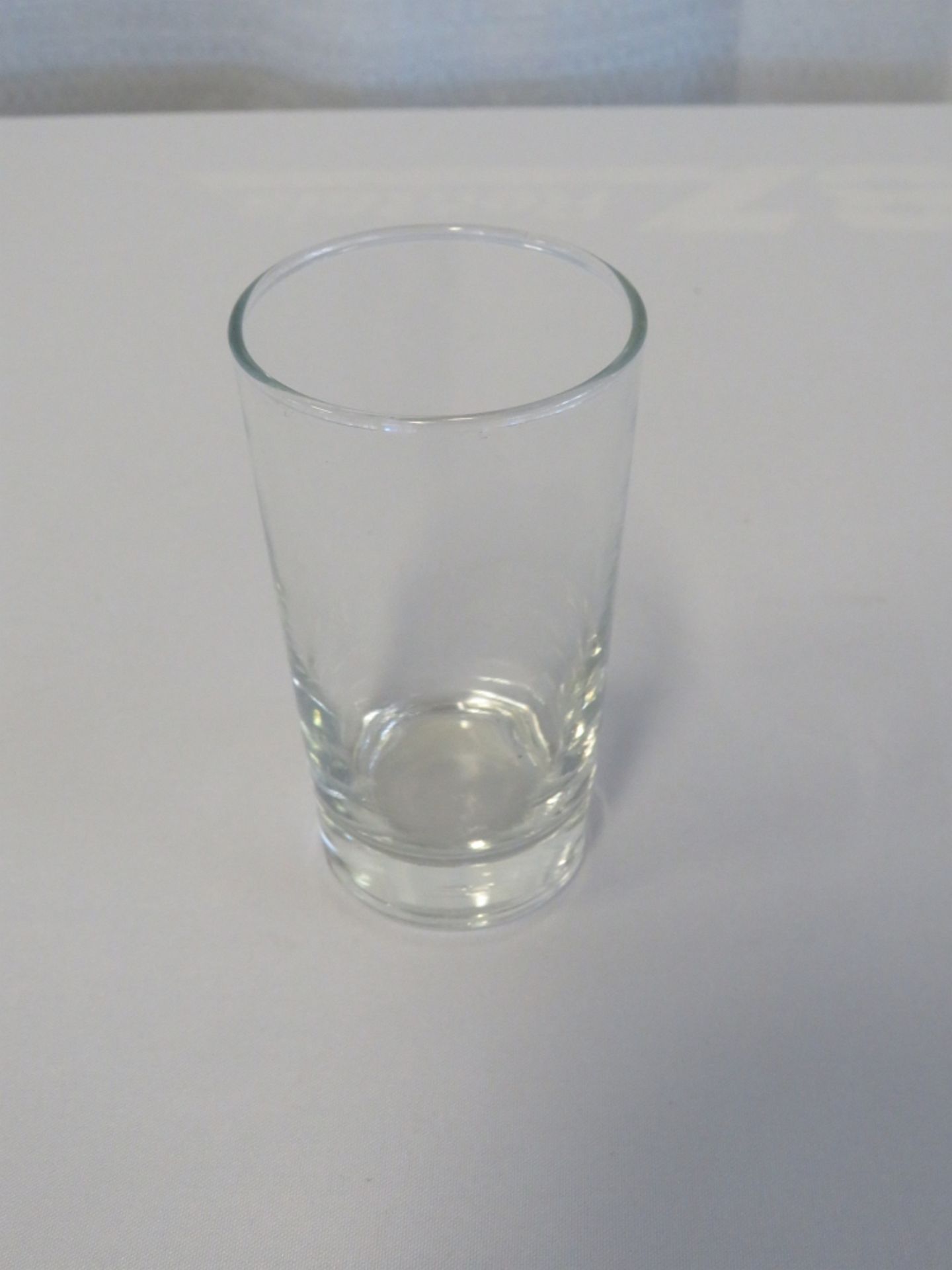The image depicts a simple, clear drinking glass placed at the center of a white table or surface, with an off-white wall visible in the background. The glass, likely intended for water and capable of holding about eight ounces, features a thick bottom and a cylindrical shape that slightly bows outward towards the top. It is entirely empty and clean, with noticeable reflections of light, suggesting it may be unused or recently unboxed. The photograph is of moderate resolution and the scene appears to be set in a home, possibly in a kitchen, or in a restaurant setting awaiting use. The overall composition includes only the clear glass, the white table, and the off-white wall, highlighted by their unblemished simplicity and minimalistic aesthetic.